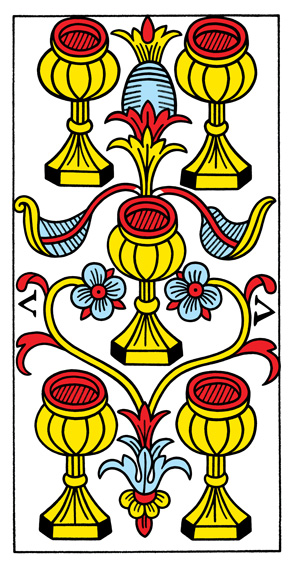The image is a meticulously crafted art piece resembling traditional tattoo artistry, characterized by its bold black outlines and solid colors. It features five chalice-shaped trophies, arranged in a distinctive 2-1-2 formation: two at the top, one centrally positioned, and two at the bottom. Each chalice is predominantly yellow with striking red circular tops. Complementing the chalices are intricate curved line designs that add fluidity and movement to the composition. 

Flanking the chalices are two vibrant blue flowers, each boasting four light blue petals with red centers. Three red leaves subtly peek out from beneath these flowers, adding to the color contrast. The flowers possess yellow stems that elegantly curve outward towards the edges of the image before turning inward, converging at the midpoint adorned with red and light blue detailing.

Additionally, the composition is framed by the letter 'V' positioned sideways on both the left and right edges, each ‘V’ pointing outward from the center, adding a symmetrical balance to the overall piece.